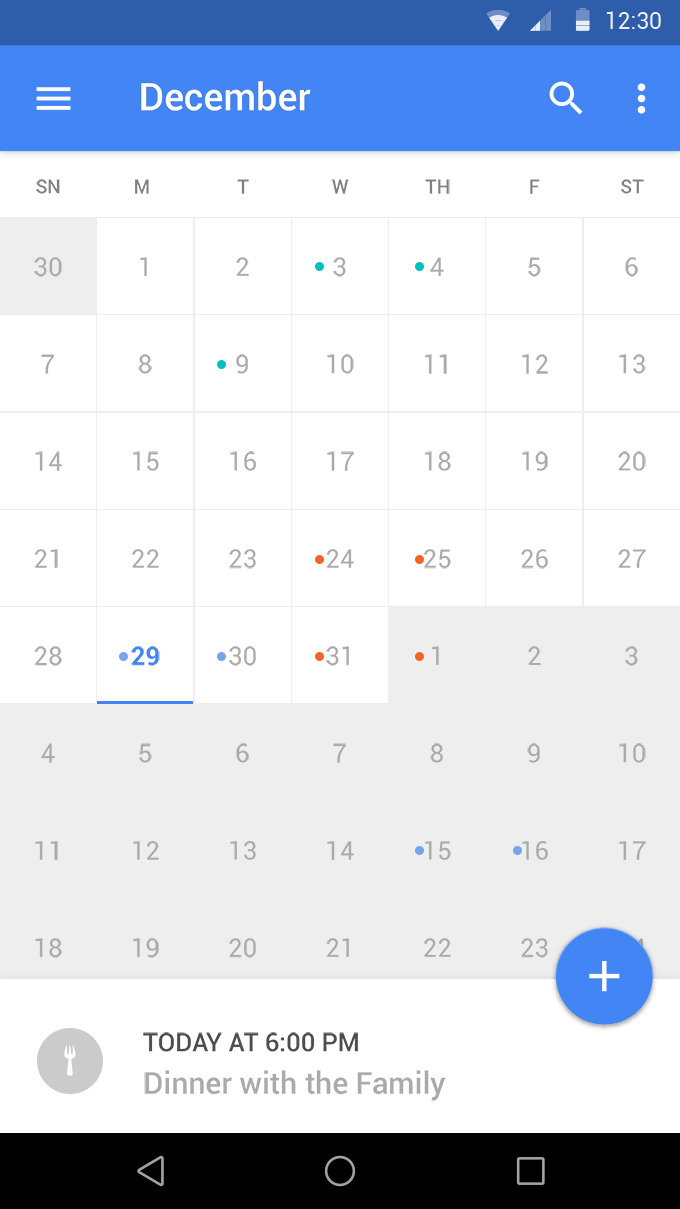A detailed screenshot of a smartphone displaying a calendar application is provided. At the top, a very dark blue banner features three out of four signal strength bars on a Wi-Fi symbol. On the right of this banner, a triangular Wi-Fi icon shows two bars, and the battery icon appears to be at around 40%. The current time is indicated as 12:30 in white text. Below this, a lighter blue, thicker bar contains three horizontal white lines stacked atop each other on the left, and the word "December" in large, bolded white letters at the center. Adjacent to "December" on the right is a white search magnifying glass icon and a vertical ellipsis (three dots stacked vertically).

The main body of the screenshot features a standard white calendar grid starting with the Sunday of the previous month, November, displaying the 30th in a darker gray, indicating it's selected or highlighted. The days of the week—Sunday through Saturday—are listed horizontally. Calendar dates of interest are marked with dots: blue dots appear on the 3rd, 4th, 9th, 29th, and 30th, likely indicating scheduled appointments, while red dots mark significant dates on the 24th, 25th, 31st, and January 1st. The transition to January is marked with a slightly grayed background from the 1st to the 24th, highlighting future dates. 

In the bottom right corner of this section, a blue dot with a white plus sign suggests an option to add a new event. Beneath the calendar on the left side, a gray circle with a white fork icon indicates an event, "Today at 6 p.m.: Dinner with the family." 

Finally, at the bottom of the screenshot is the smartphone's navigation bar, consisting of a left-pointing triangle on the left, a white circle in the center, and a white square on the right, facilitating user navigation within the phone's interface.